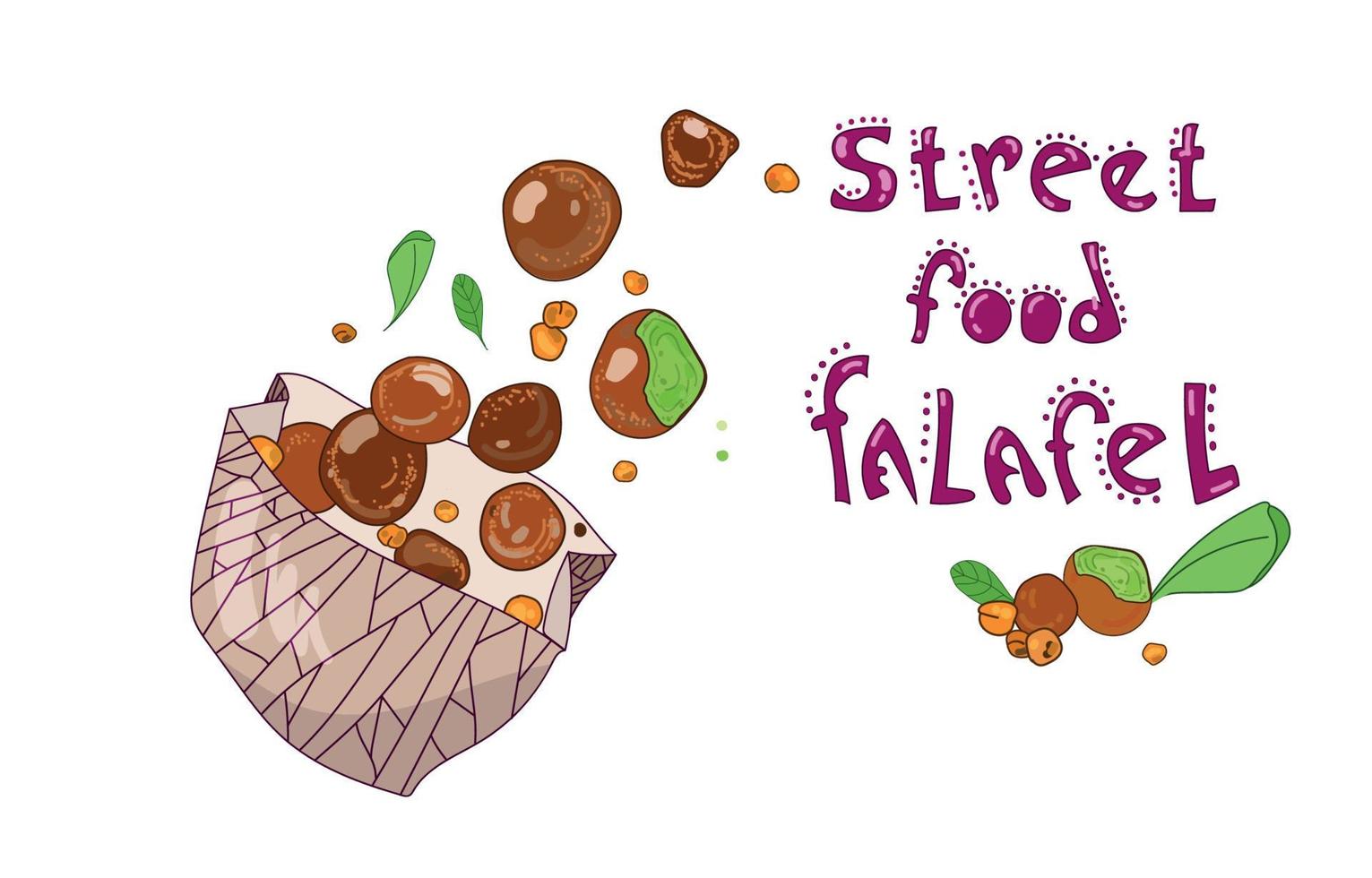This digital artwork presents a whimsical depiction under a blank white background, dominated by a playful, stylized purple text in the upper right corner, reading "Street Food Falafel." The captivating, curved font is adorned with charming dots, creating a vibrant, informal, almost child-like aura. Below this text, intricately drawn falafel pieces, chickpeas, and two green leaves are artfully arranged. A prominent falafel piece on the right shows a bite taken out of it, revealing its green interior, suggesting a savory, herb-filled treat.

On the left half of the image, a gray paper bag with a geometric design releases a cascade of falafels, chickpeas, and additional green leaves, all levitating upwards as if magically floating. This imaginative scene is clearly not photorealistic, enhancing its playful and friendly tone, which may very well serve as an enticing advertisement for a vegan-friendly or vegetarian-friendly street food vendor.